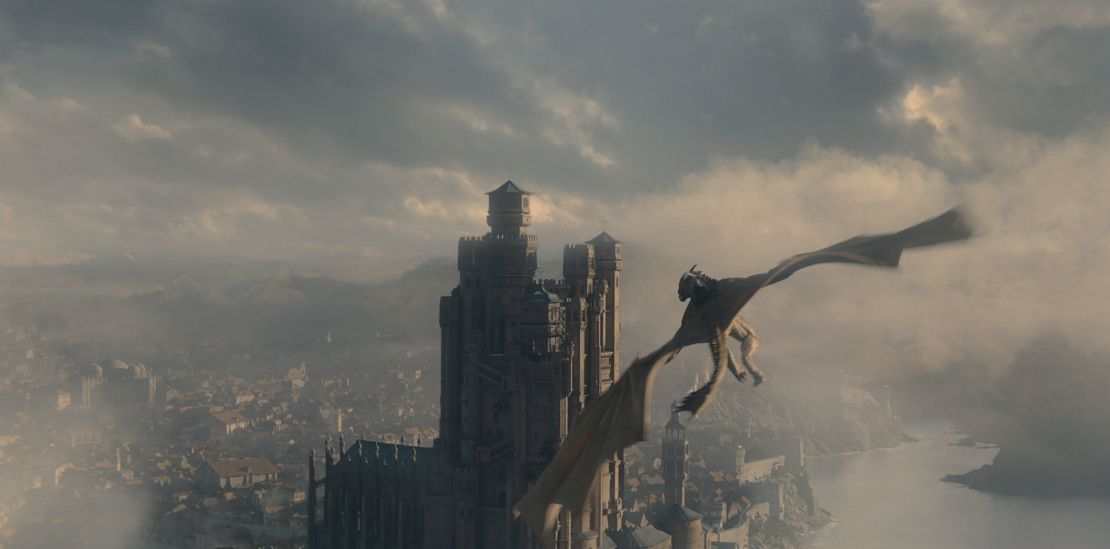This detailed, wide landscape-format shot captures a high-fantasy scene reminiscent of "The Lord of the Rings" or "Game of Thrones." The image, likely computer-generated, presents a dramatic aerial view. Central to the scene is a vast and towering medieval-style castle made of brown stone with multiple turrets sporting blue roofs. The imposing structure is nestled amidst a foggy village filled with various buildings, including a distinctive church spire. Swirls of dark, stormy clouds enshroud the village, adding to its mysterious allure.

Strikingly, a massive dragon, gray or light brown in color, dominates the foreground. The dragon, with its impressive wings spread wide, muscles tensed, and a long, fan-tipped tail trailing behind, flies away from the camera towards the majestic castle. Details like horns on its head and three spiny structures in its thin, expansive wings enhance the creature's menacing appearance. The dragon's altitude, approximately 300 feet, affords a clear view over the foggy terrain below.

To the right of the village, a river snakes into the misty distance, possibly leading to the ocean hinted at the image's lower right. The scene is set against a backdrop of rolling hills and distant mountains, all partially obscured by mist and cloud, which add depth and a touch of ethereal wonder to the image.